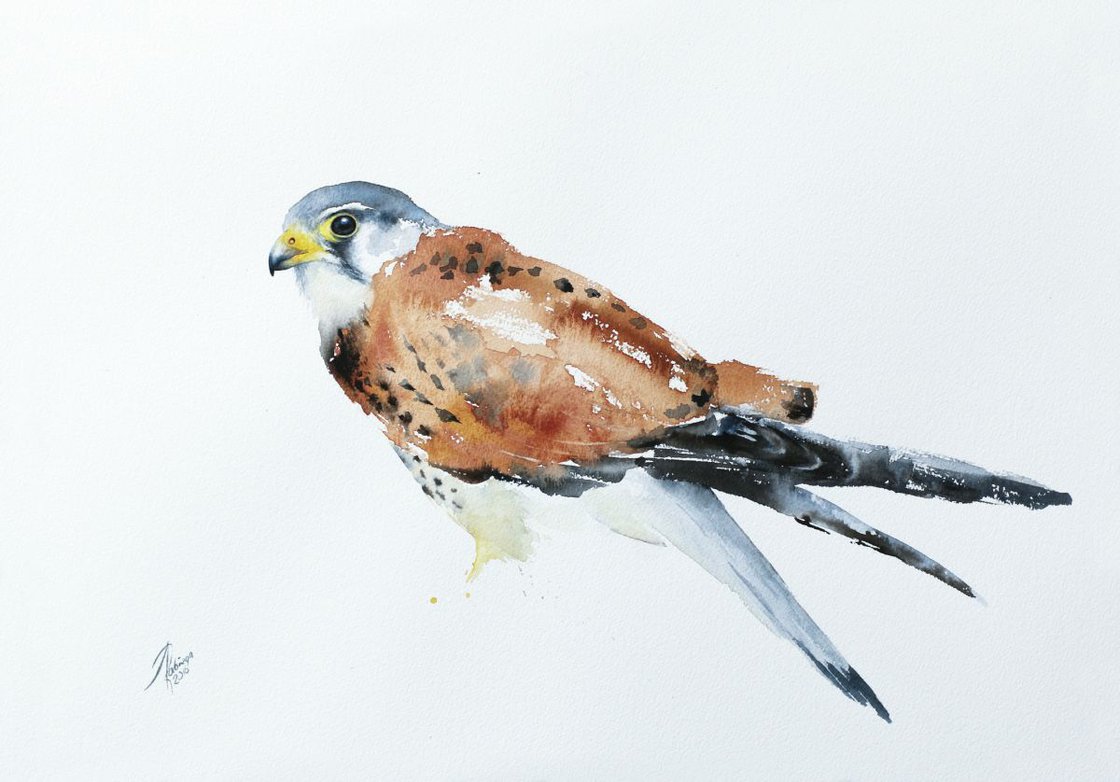This horizontal rectangular image is a detailed watercolor painting of a bird set against a white backdrop. The bird, displayed in a broadside, left-facing profile, features a striking array of colors. Its head is primarily a grayish-blue with a distinctive white line above its black eye and a yellow tinge around the front part of the eye. The beak is predominantly orange, transitioning to dark at the tip. The bird's throat and the side of its face are white, blending into a brown body speckled with black. The neck is white, the chest showcases a mix of brown and black, while the legs are white with black specks. The tail feathers, positioned towards the lower right of the image, are a blend of dark black, gray, and white, tapering to a point. Notably, the artist's signature or initials, though unreadable, are present in the bottom left corner, adding a touch of authenticity to the artwork.